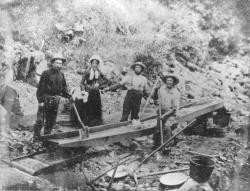This vintage black and white photograph, likely taken during the mid-1800s gold rush era, captures a group of four miners working diligently at a gold panning operation in a rocky hillside environment. The landscape-oriented image is grainy yet detailed enough to depict three men and one woman. The men, dressed in light shirts and dark pants with straw hats, hold shovels and stand around a wooden chute that spans the image from the bottom left to the mid-center. The chute has water running through it, flowing from a mostly unseen stream at the top right, to a tray underneath on the left, where the ripples indicate ongoing panning activity. The woman, positioned centrally among the three men, wears a long dress and a distinctive white bonnet with ties hanging below her chin. She is the only one without a shovel. The setting features shrubbery, mountains, and rocks in the background, adding to the sense of an outdoor, rugged mining area. Additional tools like pails, rakes, and a round black bucket are scattered around, indicating a well-equipped and presumably efficient gold mining setup. Despite the challenges in making out finer details due to the photograph’s age and graininess, the image vividly documents a moment in gold mining history.